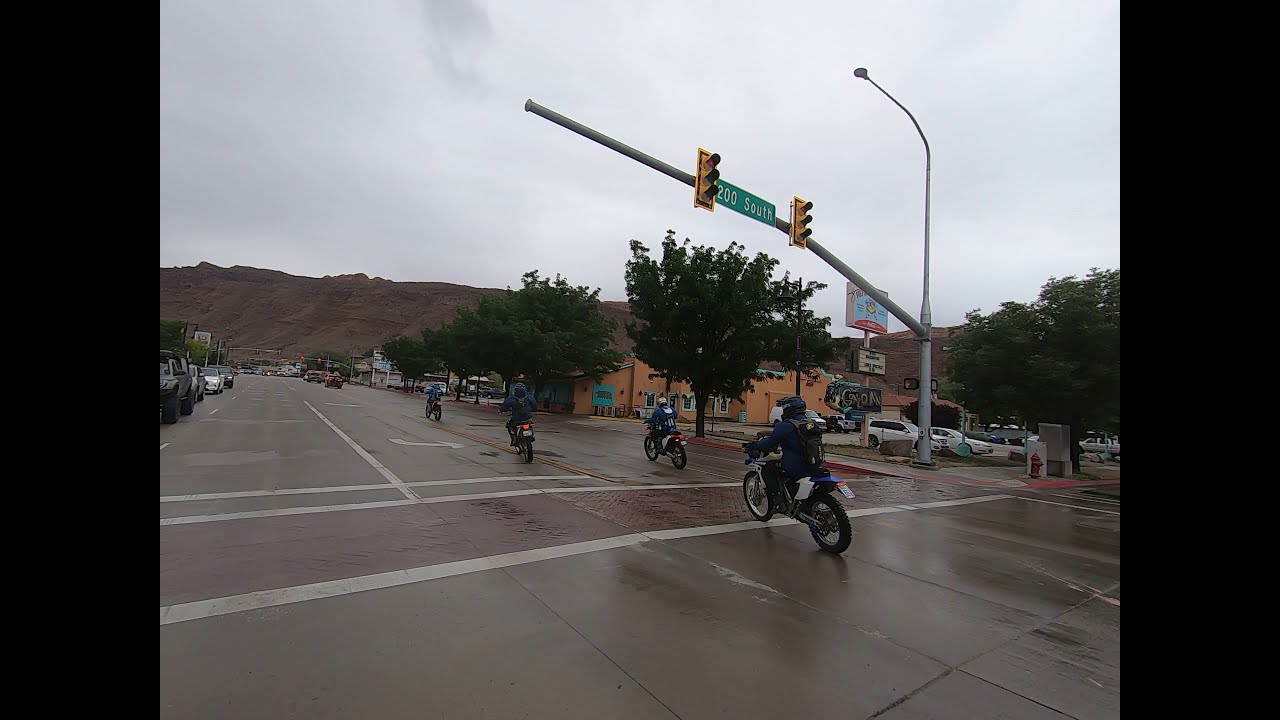The image depicts a busy daytime scene on a main road identified by a green sign that reads "200 South" in white font, positioned between two yellow traffic lights on a horizontal bar atop a traffic light pole. The road appears wet, indicating recent rain, and features a red brick crosswalk beneath the traffic lights. Four motorbikes are traveling through the intersection, amidst several cars parked along the sidewalk, which is lined with multiple trees. In the background, an orange building with a blue billboard suggests a commercial area, possibly housing a fast-food restaurant. The sky is completely overcast with gray clouds, casting a gloomy light over the scene. A brown, rocky mountain range is visible in the distance, adding to the outdoor setting's natural elements. The image has long vertical black lines framing it on the left and right sides.